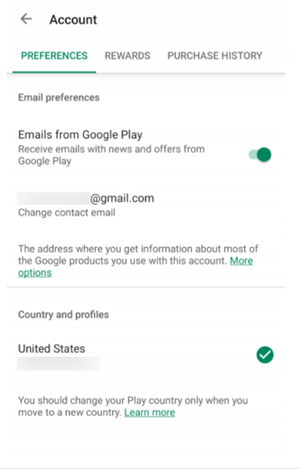In the upper left corner of the image, there is a text label that reads "Account" in black font on a white background. Below this, across the top of the page, there are several tabs: "Preferences," "Rewards," and "Purchase History." These tabs are all written in black, except for "Preferences," which is highlighted in green and underlined in the same color.

Under the "Preferences" tab, the first section is labeled "Email preferences." Directly beneath this is the subheading "Emails from Google Play," followed by the text, "Receive emails with news and offers from Google Play." To the right of this line, a switch toggle—colored green to indicate it is turned on—is visible.

Further down, on the left side, an email address is listed as "sgmail.com," although it is partially concealed with a grey overlay. Below the email, the option "Change contact email" is presented. A descriptive note follows, explaining, "The address where you get information about most of the Google products you use with this account." The phrase "More options" is highlighted in green at the end of this note.

Continuing down the left side, another section titled "Country and profiles" appears, indicating the United States, although the exact location is obscured in grey. Adjacent to this, on the right side, there is a green checkbox with a white checkmark inside it.

At the bottom of this section, advice is given: "You should change your Play country only when you move to a new country." A "Learn more" button, highlighted in green, is positioned at the bottom.